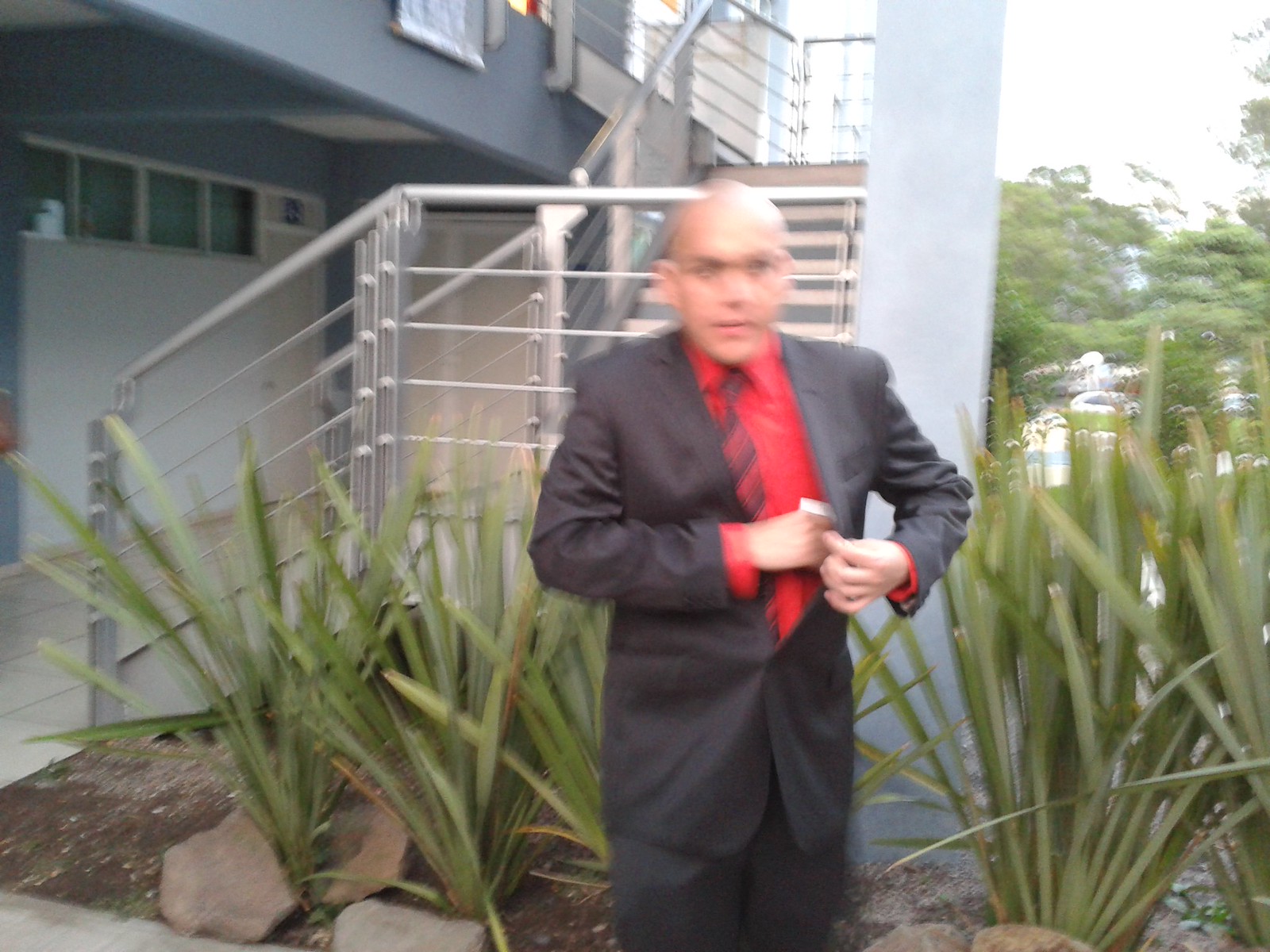The image features a Caucasian male dressed in a gray suit paired with a red collared dress shirt and a red and black necktie. He is bald and appears slightly blurred in the photograph, perhaps due to motion or focus issues. The man is using his right hand to place what seems to be a piece of paper into the interior pocket of his suit jacket. He is positioned in front of an elegant house, which resembles a vacation home or resort. The background is adorned with tall leafy plants and a stretch of exposed soil or dirt. Prominent white rock boulders also contribute to the picturesque setting.